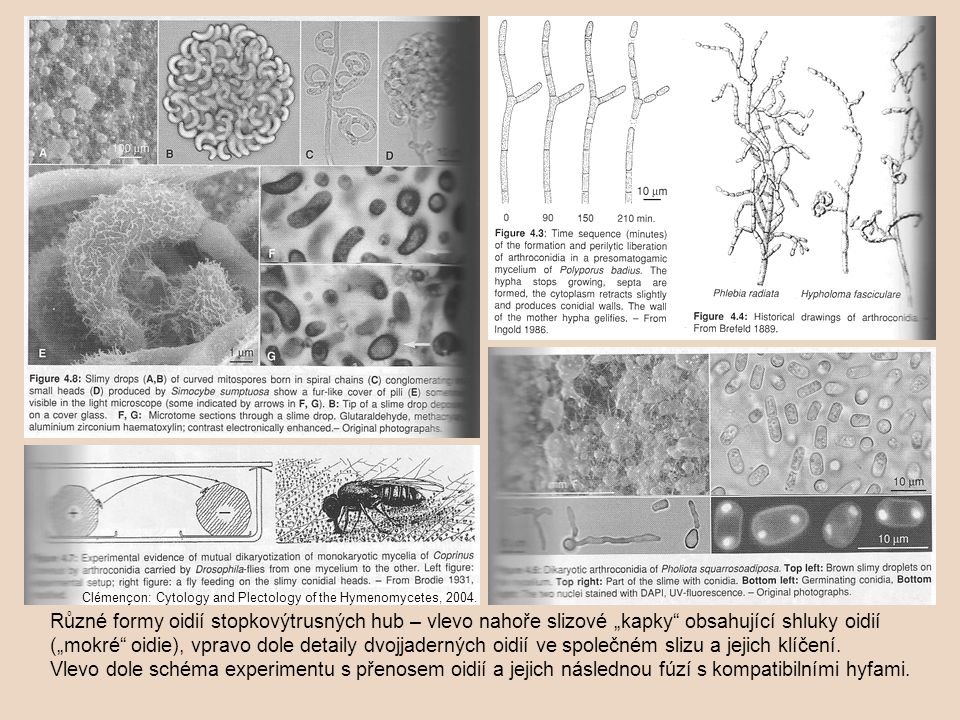The image is a scanned double-page spread from a scientific book, featuring detailed studies of bacteria and microorganisms. The left page predominantly displays seven natural images of bacteria and microorganisms arranged in a grid, each accompanied by descriptive text labeled as figure 4.8. Below this grid is an illustration labeled as figure 4.7, depicting experimental evidence of mutual dekaryotization of monokaryotic mycelia of Coprinus, though this portion appears slightly faded and blurry from the scan. The illustration is annotated with the text: "Experimental evidence of mutual dekaryotization of monokaryotic mycelia of Coprinus," along with a date and reference to Clement's cytological and plectological studies of the Hymenomycetes.

The right page contains an illustration of branched microorganisms, with text indicating that these are historical drawings of Amphiroconda from Brayfield, 1889. Below this illustration, there is another scanned image of microorganisms viewed under a microscope, accompanied by black text in a non-English language, likely Spanish, against a beige background. The detailed descriptions and various illustrations suggest the book is a comprehensive scientific reference in microbiology or cytology, with the content emphasizing the study and historical documentation of microscopic life forms.